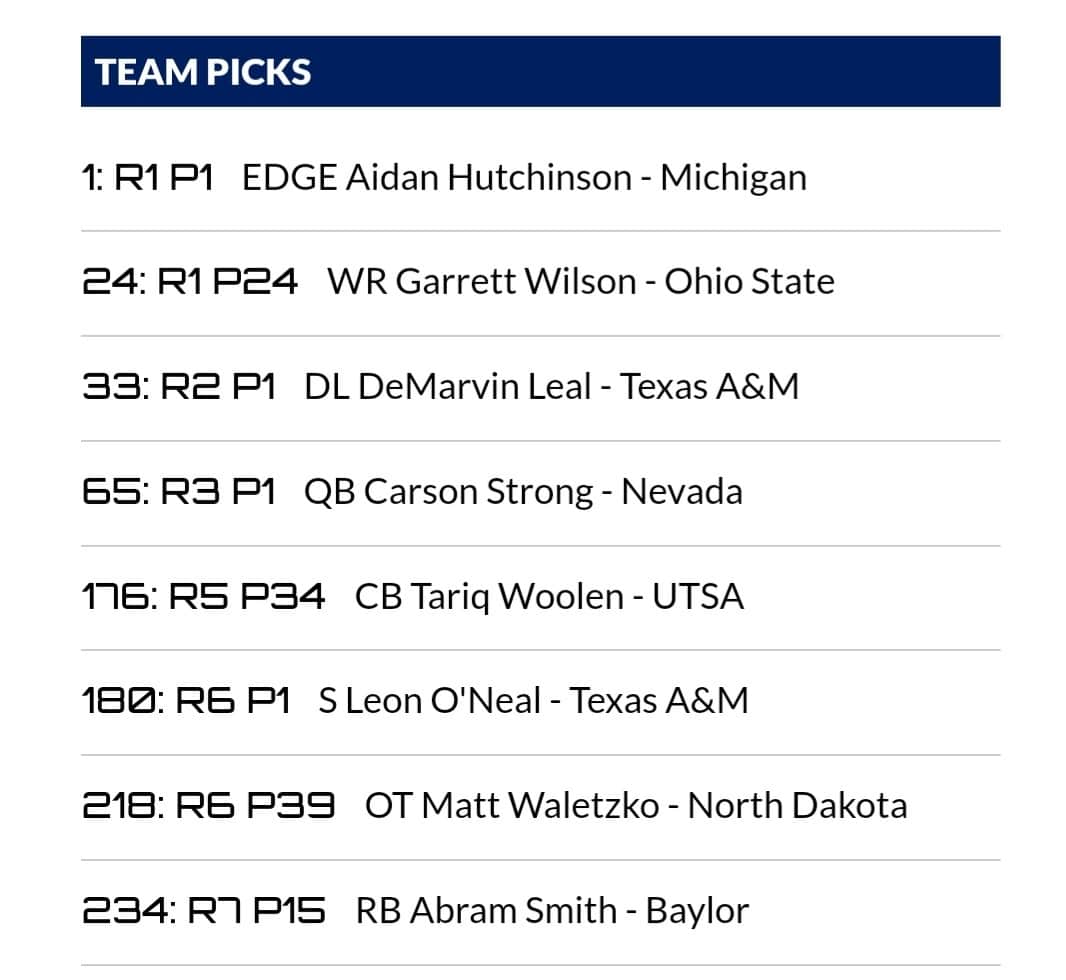The image features a dark blue banner at the very top with the text "Team Picks" written in white. Below the banner, there are several segments of text, each separated by thin gray or green lines:

1. Immediately below the banner, there is the text "1R1P1, Edge, Aiden Hutchinson, Michigan" written in dark blue.
   
2. Following a thin light gray line, the text reads "24R1P24, WR, Garrett Wilson, Ohio State."

3. Another thin gray line separates the next segment, which displays "33R2P1, DL, DeMarvin Leal, Texas A&M."

4. Below yet another thin gray line is the text "65R3P1, QB, Carson Strong, Nevada."

5. After an additional thin gray line, it reads "176R5P34, CB, Tariq Woolin, UTSA."

6. A thin green line then divides the next segment, which says "180R6P1, S, Leon O'Neal, Texas A&M," followed by another thin gray line.

This structured layout appears to represent selections or picks, potentially for a draft or similar event, with specific references to the player's position, name, and school.